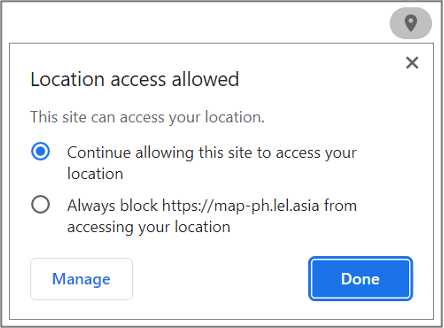Detailed Caption:

An image depicts a pop-up notification on a smartphone screen. The background of the screen is entirely white. In the top right corner, there is a small gray circle containing a location symbol, which is shaped like an upside-down teardrop with a dot in the center.

Beneath the circle, a box with a lighter border appears. At the top left of this box, bold text reads "Location access allowed." Directly to the right of this text, an 'X' symbol is situated in the top right corner of the box.

The second line within the box states, "This site can access your location." On the third line, there is a small circle with a blue dot in the middle followed by text that reads, "Continue allowing this site to access your location."

On the next line, there is another circle, this one empty, beside the text: "Always block https://map-ph.lel.asia from accessing your location."

At the bottom left of the box, the word "Manage" appears in blue text, while on the bottom right, there is a blue button labeled "Done."